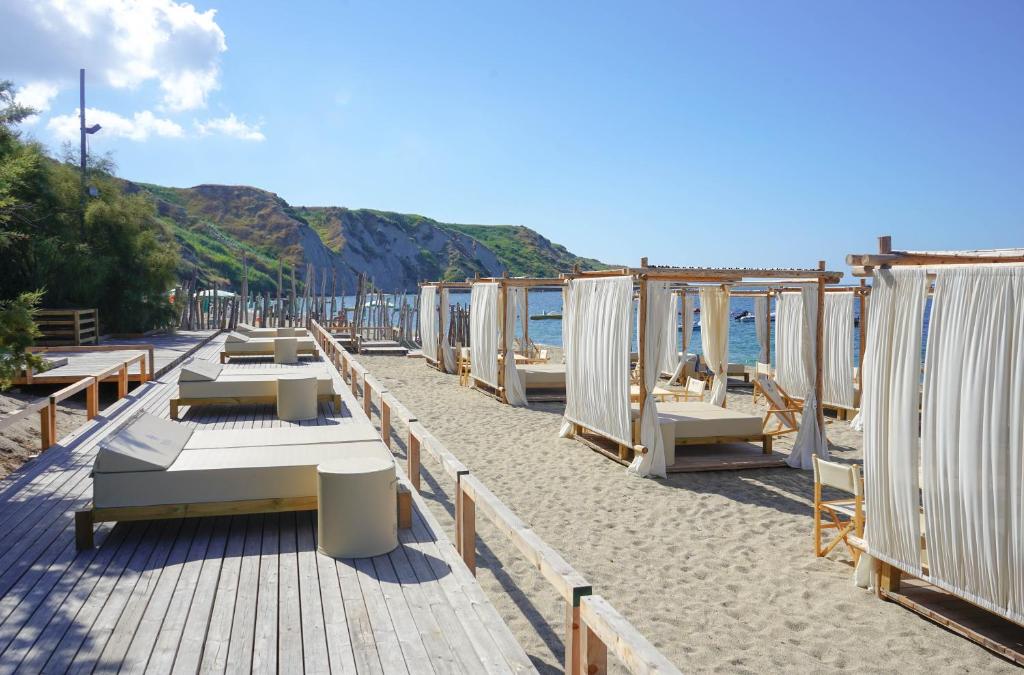The photograph captures a beautiful beach scene at a luxury resort. In the foreground, there is a wooden deck with railings, arrayed with beige lounge beds where guests can relax. Extending beyond the deck, the sandy shore is dotted with multiple covered lounging areas that resemble Cleopatra-style compartments, with wooden bases and white draping sheets that create cozy, private spaces. These lounging areas blend seamlessly into the sandy beach, adding to the serene ambiance. Alongside the shore, the vibrant blue waters of the ocean are visible, dotted with swimmers enjoying the waves. In the distance, towering, grass-covered mountains provide a stunning backdrop under a mostly clear blue sky with some patches of white clouds on the left. The atmosphere is distinctly tropical and exudes an air of opulence and relaxation.